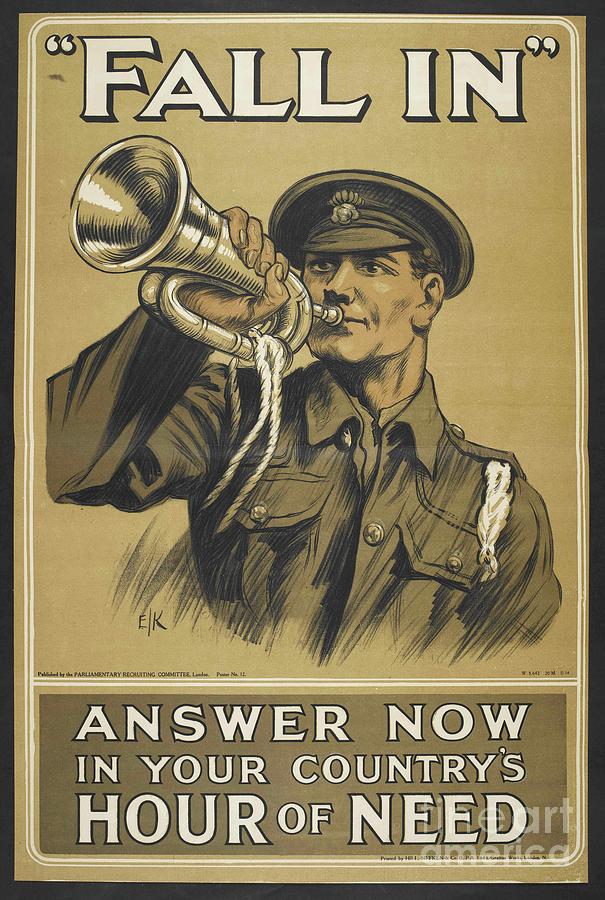This vintage army recruitment poster, possibly from World War I or World War II, features a detailed illustration rather than a photograph. The poster is bordered in black with a second white double-line border framing a tan background. At the top, in bold white text outlined in black, it reads "Fall in." Dominating the center, a soldier in a dark green military uniform is depicted blowing a bugle adorned with ropes and a white tassel. He wears a hat as part of his uniform and has a distinctive white feather on his left shoulder. At the bottom of the poster, within a separate box, the text urges, "Answer now in your country's hour of need." The artwork is signed with the initials "E/K" on the left side, possibly attributed to the artist. Additionally, there is a Fine Art America watermark at the bottom, suggesting the image has been reproduced for modern distribution.